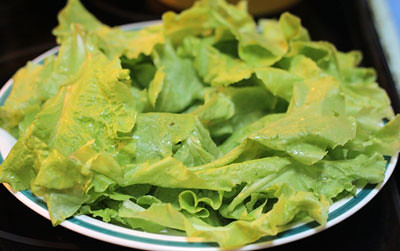This is a close-up photograph of a white plate with an aquamarine rim, set against a very dark, blurred background. The plate, which dominates the image, is piled high with freshly washed romaine lettuce, displaying a rich variety of green shades from light to dark, with occasional highlights where the light hits the leaves, giving them a yellowish tinge. There are visible water droplets or possibly a light, oily dressing glistening on the leaves under the light. The dark brown surface beneath the plate contrasts sharply with the vibrant greens, emphasizing the freshness and simplicity of the salad. The plate appears to be about eight inches in diameter and is filled entirely with plain lettuce leaves, stacked a couple of inches high. No other ingredients or text are present in the image, maintaining a clear focus on the fresh, green lettuce.